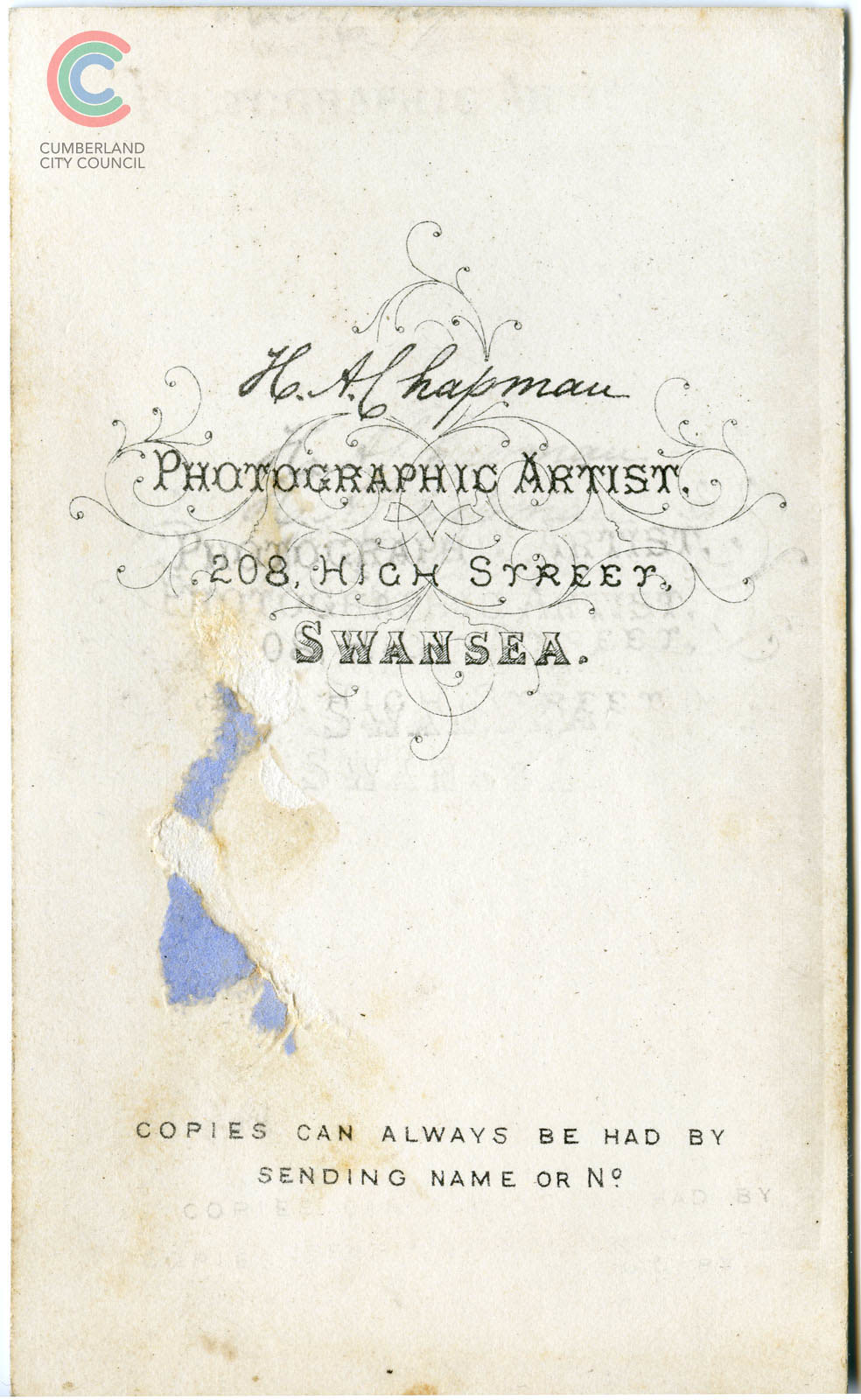The image appears to be the front page of an old advertisement or pamphlet, distinguished by its weathered, off-white paper showing signs of foxing, staining, and slight blue paper residue on the center-left. In the top left corner, there's the emblem of the Cumberland City Council, composed of three nested C's in descending size: a red C, followed by a green, and then a blue C. The center of the image features an ornate, cursive script reading "H.A. Chapman, Photographic Artist, 208 High Street, Swansea," over a decorative, curving filigree design with two drops of blue and gold. Below this, in an all-caps black font, it reads, "Copies can always be had by sending name or N.O.," with "NO" superscripted with an "O" and underlined.